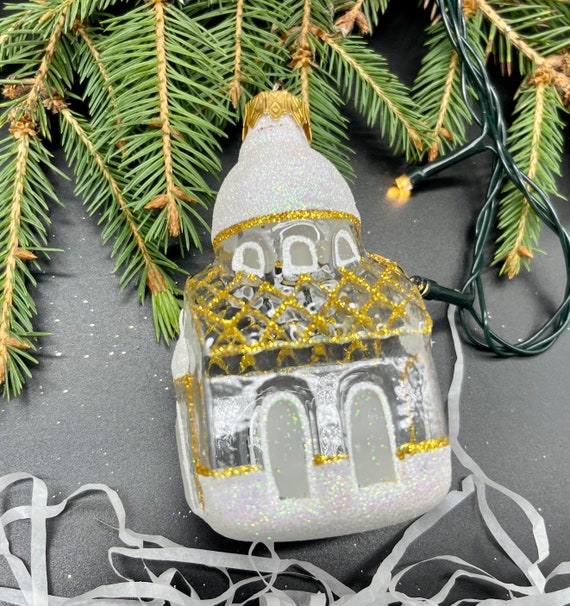The image is a vertical, rectangular close-up of a Christmas ornament. The ornament is designed to resemble a tiny, frosted house or a miniature church, complete with a square base, a golden roof, and a cupola ending in a gold hook at the top. It lies on a gray, grainy surface, possibly a table, which is sprinkled with white grains that might be artificial snow. Above the ornament, green pine tree branches can be seen, suggesting the presence of a Christmas tree. Black cables, likely for Christmas lights, drape alongside the ornament. Additionally, there are torn pieces of white paper or ribbons under the ornament, adding to the festive display.